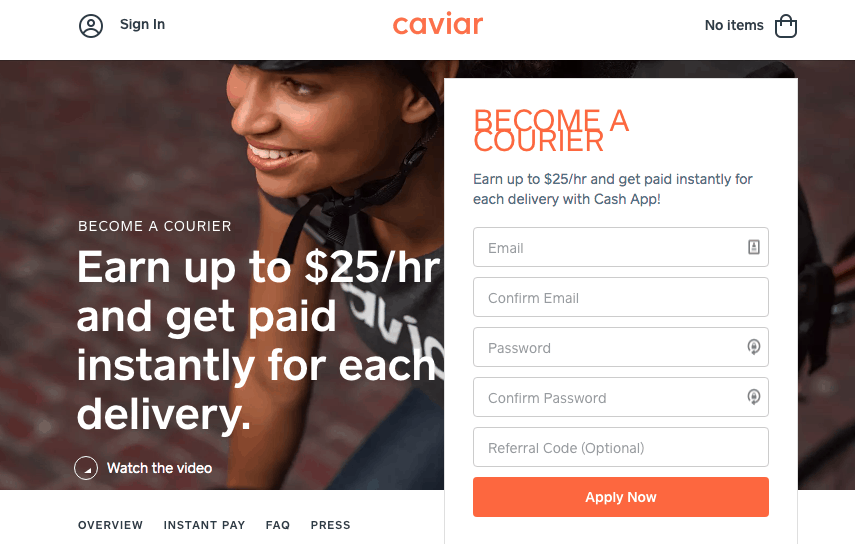In the center, displayed in vibrant orange text, is the word "CAVIAR." To the left, there is a clickable "Sign In" option in black text. On the right side, the text "No Items" is shown alongside an image of a shopping bag. Below this header, a smiling woman with tan skin is featured prominently. She is wearing a bicycle helmet and is seated on a bike. She is dressed in a gray tank top with white text on it, paired with gray leggings. The accompanying text reads, "Become a COURIER. Earn up to $25 an hour and get paid instantly for each delivery." Positioned beside a white circle that invites users to "Watch the video."

To the right of the image, there is a section inviting individuals to "Become a courier." It further explains, "Earn up to $25 an hour and get paid instantly for each delivery with Cash App." Below this message, there are fields for entering an email address, confirming the email, creating a password, confirming the password, and inputting a referral code. At the bottom, an orange button labeled "Apply Now" is visible.

In the bottom left corner, all in uppercase letters, there are navigational choices: "OVERVIEW," "INSTANT PAY," "FAQ," and "PRESS."